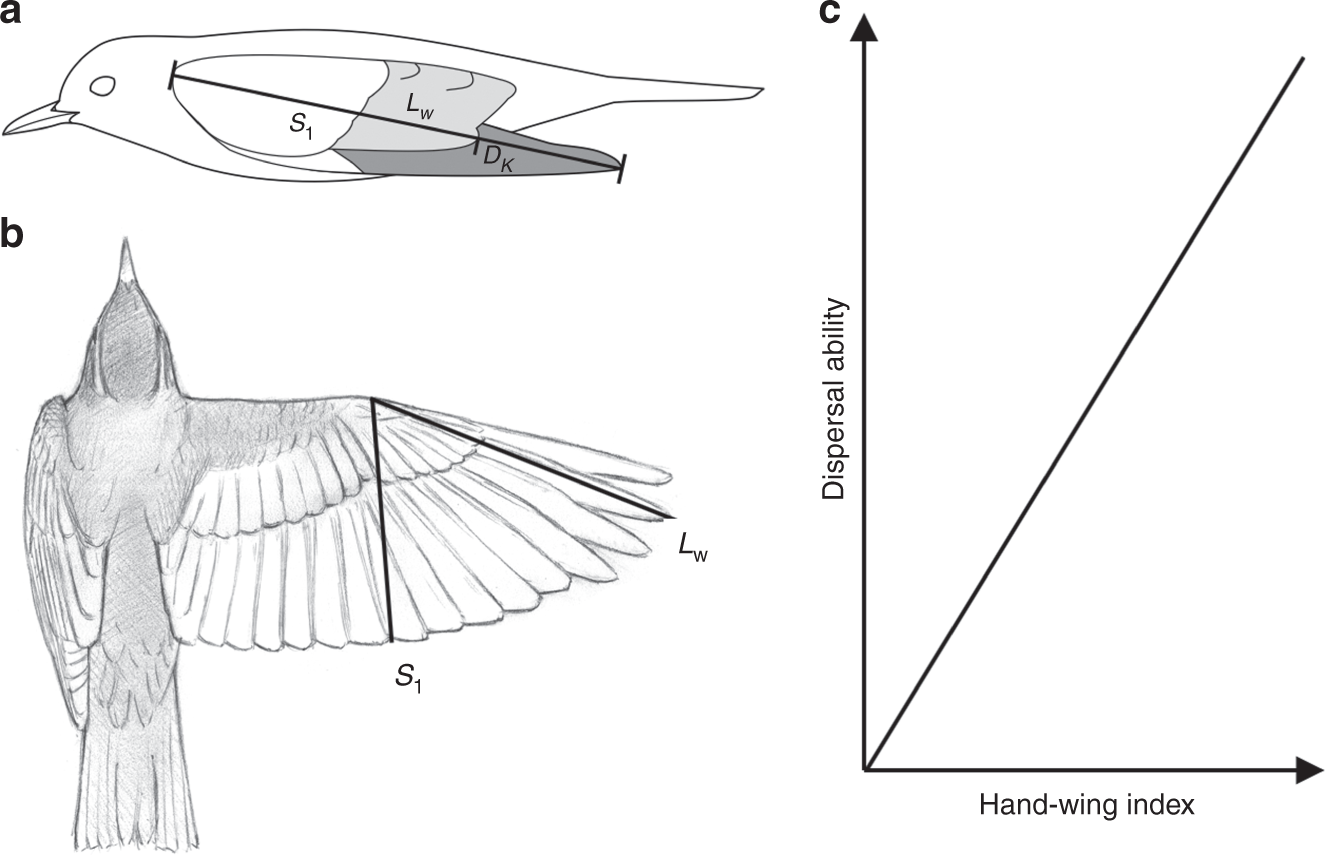The image consists of three detailed diagrams labeled A, B, and C, depicting different aspects of a bird and a related graph. Diagram A, located at the top left, is a side view of a bird featuring an outline-only design. The bird is facing left with its head towards the left and tail towards the right. This diagram is sectioned internally into three parts: the front section is white and labeled S1, the middle section is gray with the label LW, and the back section is black labeled DK. The insides are simplistic, traced in black with a visible center line indicating wing distance. Below this, Diagram B demonstrates an overhead view of a bird in flight; its head is at the top, tail at the bottom, with the left wing closed and the right wing open. This diagram utilizes grayish-black shading and white wings, including a triangle-like pattern near the wing tips with similar labels. Diagram C, positioned to the right, is a line graph that shows the relationship between "Dispersal Ability" on the y-axis and "Hand-Wing Index" on the x-axis, represented by a line running upwards to the right corner, creating a 90-degree angle. All diagrams together provide a comprehensive and detailed analysis of the bird’s anatomy and flight dynamics.